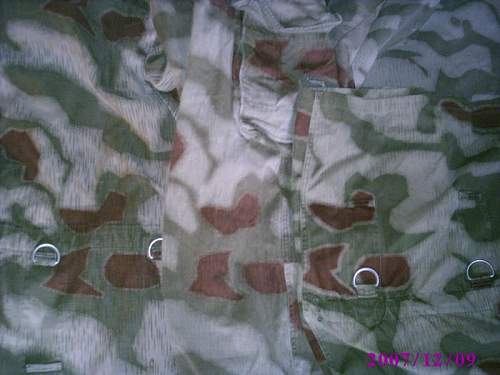This zoomed-in photo, dated 2007-12-09 as displayed in pink in the lower-right corner, captures an indistinct camouflage-patterned fabric. The fabric showcases a blend of green, gray, rust, and white, with unique red shapes resembling L’s and octagons scattered throughout. The texture reveals clear divisions between sections, suggestive of a layered or overlapping garment, perhaps a jacket or shirt. Notably, four evenly spaced loops traversing the bottom quarter from left to right hint at functional elements like buttons or clasps. Despite its ambiguous nature, the close-up nature of the photo reveals a meticulously detailed fabric surface.